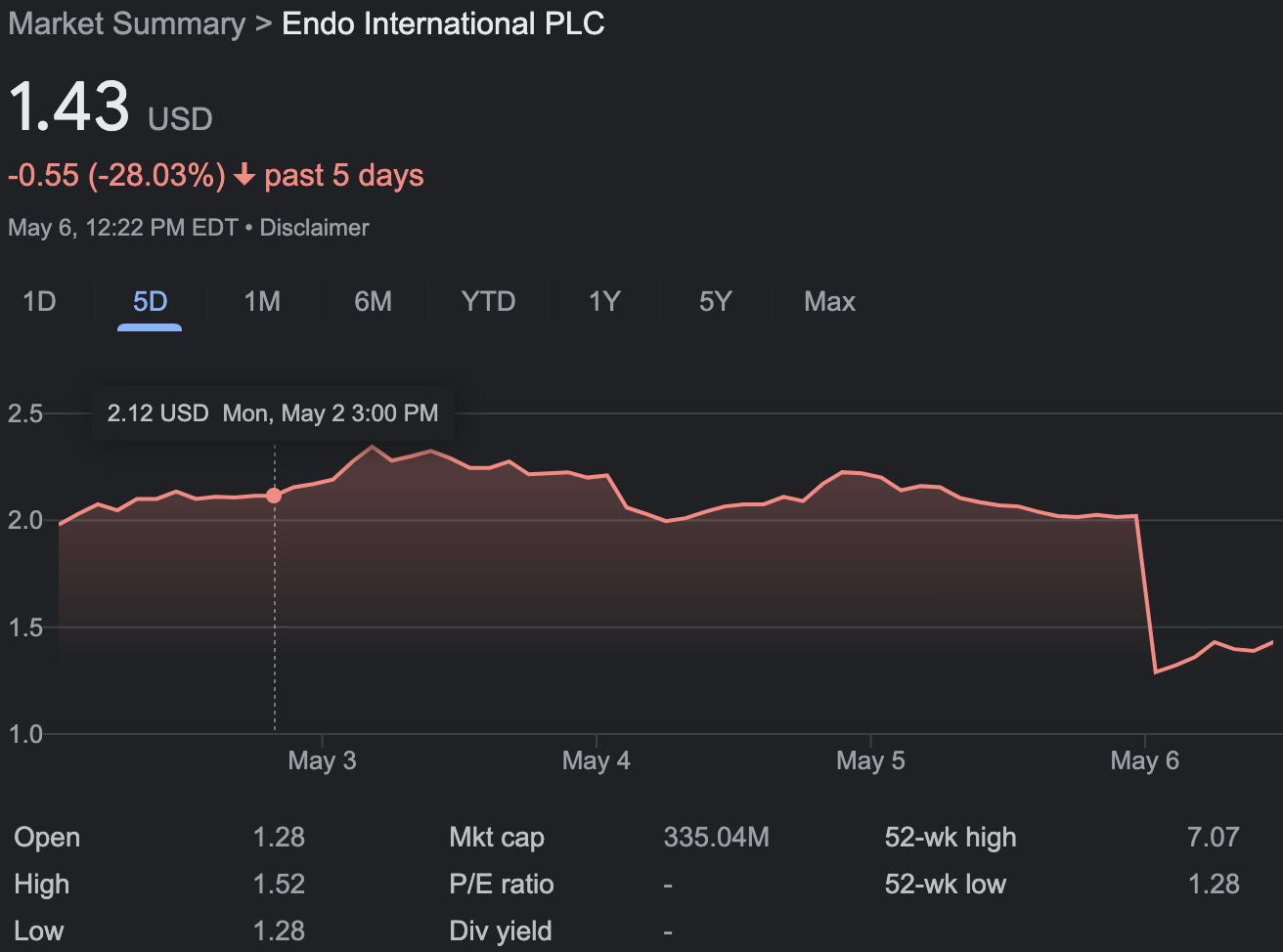This image captures a screenshot of a website displaying a financial graph for Endo International PLC. The graph features a detailed market summary, including a current stock price of 1.43 USD, with a notable decrease of 0.55 USD in the past five days. Data is timestamped for May 6th at 12:22 PM EDT. The background of the graph is characterized by pinkish lines, and regions under the line graph are highlighted in a greyish pink color, creating an illuminated effect. The peak stock price shown at the top is 2.12 USD, recorded on Monday, May 2nd at 3:00 PM. The timeline along the bottom marks important dates from May 3rd to May 6th. The graph illustrates a steady trend until a notable decline on May 6th, after which it shows a slight upward movement. There is also a visible disclaimer on the page.